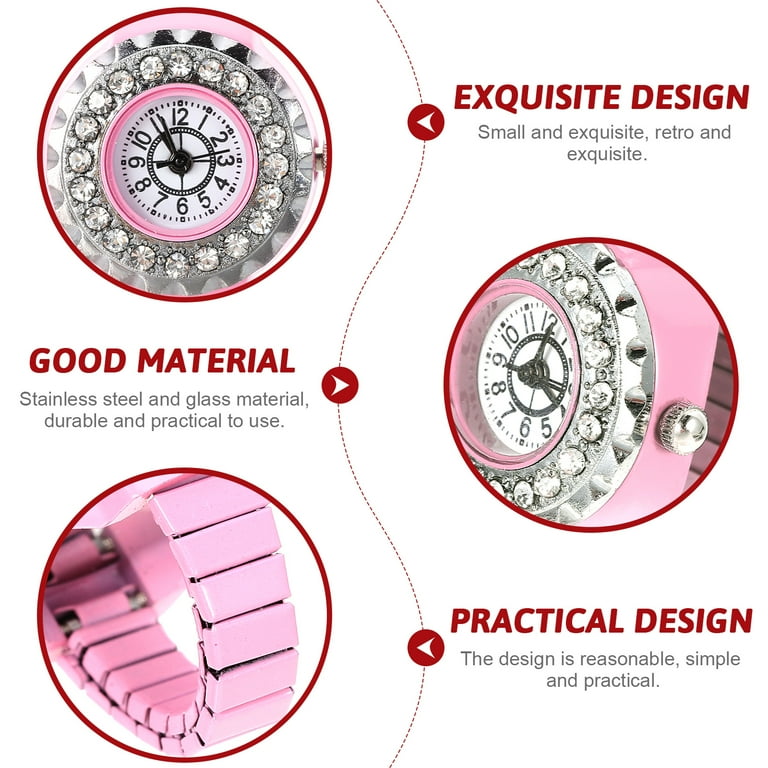The image is a detailed product advertisement for a stylish watch, featuring three distinct photographs against a white background. The first image showcases the watch face from a frontal perspective, adorned with diamond-like gems around the rim and a small pink border encircling the white dial, which features bold black numbers and hands. This section is highlighted with the caption, "Exquisite design. Small and exquisite. Retro and exquisite," emphasized in red. The second image focuses on the silver knob, complemented by the pink frame, accompanied by a caption reading, "Good material. Stainless steel and glass material. Durable and practical to use." The third image displays the pink articulated wristband of the watch, described by the caption, "Practical design. The design is reasonable, simple, and practical." This cohesive presentation underscores the watch's blend of elegance, quality materials, and practical design.